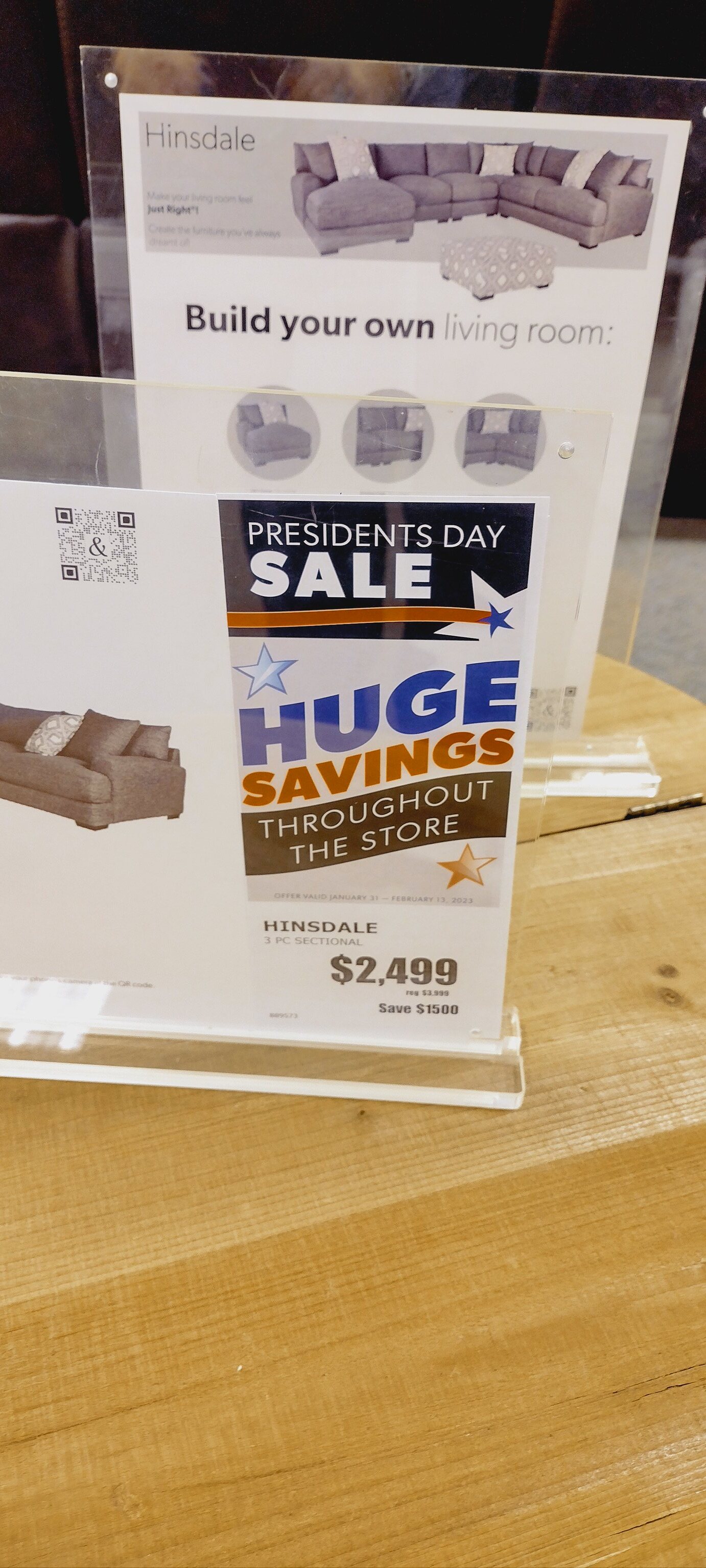In a bustling furniture store named Hinsdale, a pair of advertisement signs prominently captures shoppers' attention. The signs are encased in clear plexiglass holders, which consist of two sheets of plexiglass that sandwich the flyers securely, resting on a sturdy perpendicular base. One sign, positioned in the background, invites customers to "Build Your Own Living Room," suggesting a customizable shopping experience. The more prominent sign in the foreground entices visitors with a "Huge President's Day Sale" offering substantial savings throughout the store, highlighting a particular furniture set priced at $2,499. Each flyer integrates a QR code, indicating their modern and interactive nature, potentially leading customers to more information or exclusive online deals.